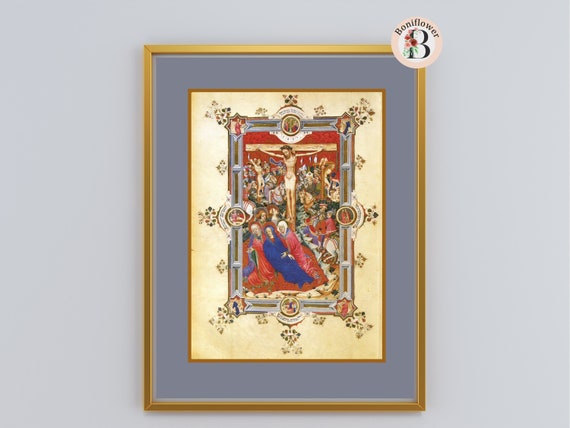The photograph showcases a richly detailed artwork in a gold frame set against a gray wall. The artwork, bordered by gray matting, portrays a medieval-style depiction of the crucifixion of Christ. The central image, resembling old paper or a scroll, is outlined in gold and set against a background of unevenly toned beige and yellow. Within the scene, Christ is nailed to a tan cross, wearing a white cloth and crowned with thorns. The red sky forms a dramatic backdrop to the image.

In the foreground, three women clad in red and blue cloaks huddle together near a red ground area that resembles a carpet. This detail is complemented by chaotic scenes in the background, where numerous figures, perhaps Roman soldiers, are in motion, and one appears to be mounted on a horse.

Additional elements of the artwork include eight distinct medallions with inscriptions, positioned at each corner and the middle points along the sides of the image, adding a layer of intricate detail to the overall composition. Despite its small size, the artwork evokes a rich tapestry of medieval iconography and poignant historical narrative.